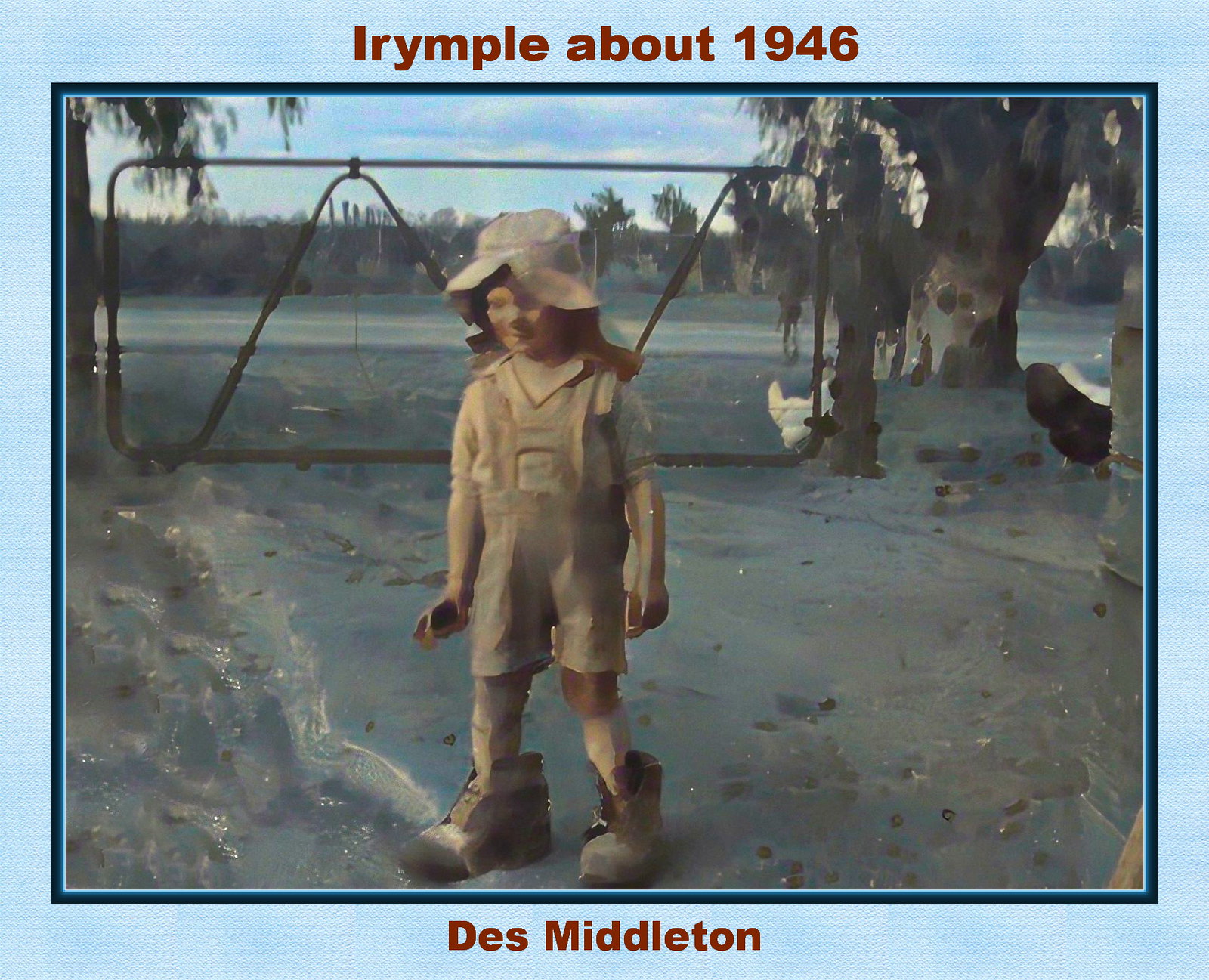The image appears to be a detailed, but somewhat blurry, color photograph with a light blue border. It depicts a small girl standing on sand or dirt near a large gate. The girl is wearing an oversized Panama-style hat in a beige or khaki color that matches her entire outfit. This includes short overalls, a t-shirt underneath, and knee-high socks, all in the same beige khaki shade. She is also wearing disproportionately large adult male boots. The girl's expression is impish and joyful, highlighted by her short brown hair. In the background, a blue sky with white clouds can be seen above trees and towers, and there are chickens by the trees. The top of the image has the inscription "Irymple about 1946," and the bottom reads "Des Middleton" in red letters.